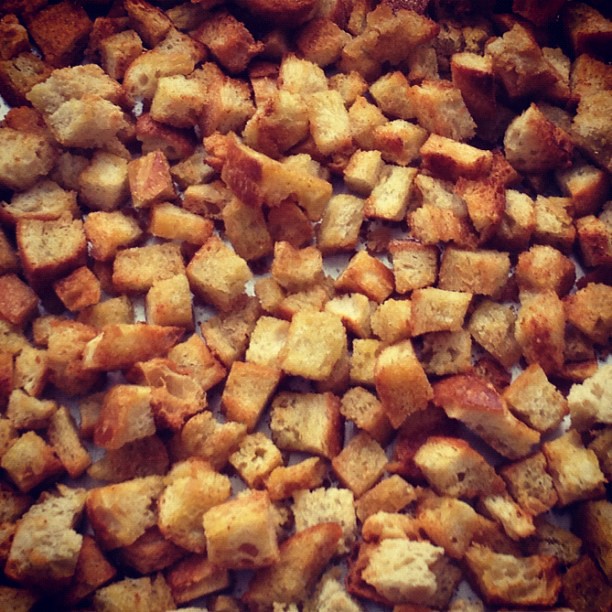This close-up image showcases a baking tray, likely stainless steel or aluminum, crowded with uniformly cubed pieces of bread. Each bread chunk is a small, thumbnail-sized piece, toasted to a crisp, golden brown color. The colors range from various shades of yellow and tan to brown and beige, indicating a well-toasted texture. The bread cubes appear to be prepared as homemade croutons, possibly for use in salads or stuffing. There are some visible crumbs scattered across the tray and layered on top of one another, suggesting they were either air-dried for a few days or baked in the oven with a drizzle of olive oil and seasonings. The trays' white parchment surface peeks through in a few spots, adding contrast to the golden hues of the bread. This image is zoomed in, filling the entire frame, making it difficult to gauge the number of bread cubes but emphasizing their texture and uniformity. No text is present in the image.